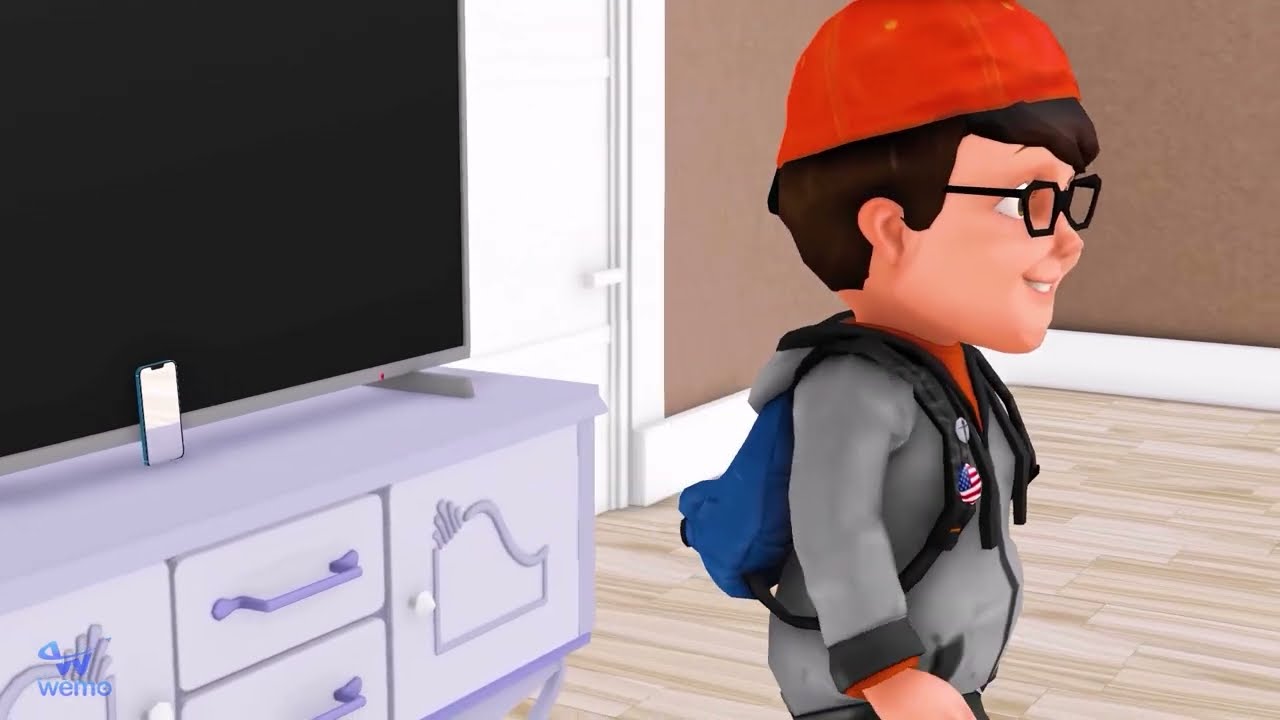This detailed caption combines all the given details:

The image appears to be from a cartoon or a video game and features a young boy standing in what looks like a bedroom. He has short dark brown hair and is wearing a backwards orange baseball cap along with black-framed glasses. His outfit includes a gray hoodie over an orange shirt and a blue backpack with black straps adorned with an American flag button pin and a cross. The boy is facing to the right, looking away from the viewer. 

The room features a light purple wall with white baseboard. In the lower left-hand corner, there is a light purple dresser with dark purple handles. On top of the dresser sits a large silver-framed TV, and a cell phone is propped up against it. To the center-left of the scene, there's a partially visible white door. 

The image style is digital art and the floor appears to be wooden. The overall color palette includes shades of orange, gray, blue, black, silver, purple, white, tan, and brown. The perspective of the image focuses on the boy from his hips to the top of his head, creating a horizontal rectangular composition.